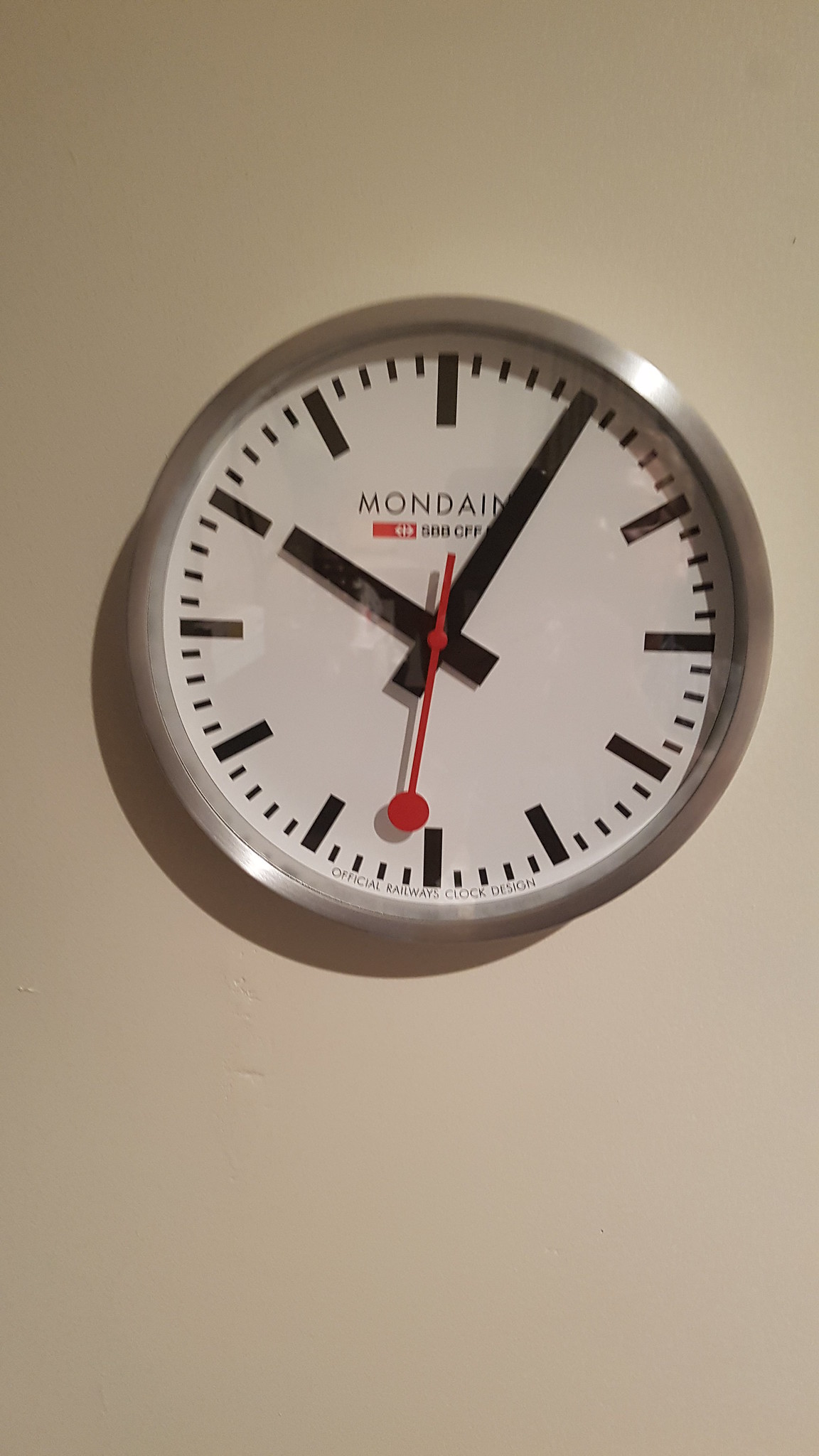The photograph captures a round analog clock mounted on an eggshell-colored wall. The silver-framed clock is styled without numerals; instead, it features thick black lines to denote the hours and smaller black lines in between for the minutes. The time displayed is 10:05, with the thick black hour and minute hands indicating this. The thin red second hand, ending in a small circle, is positioned at 31 seconds, between the 6 and 7 markers. Above the center of the clock face, in thin black Arial font, is the brand name "MONDAME." Directly below this, a small red rectangle contains additional black print, possibly reading "588CFF," with three white symbols inside the logo. The clock face has a tan or white backdrop, and the overall image appears slightly out of focus, with muted colors possibly due to a filter. The silver frame catches the light at the upper right and lower left sections, suggesting indoor lighting.